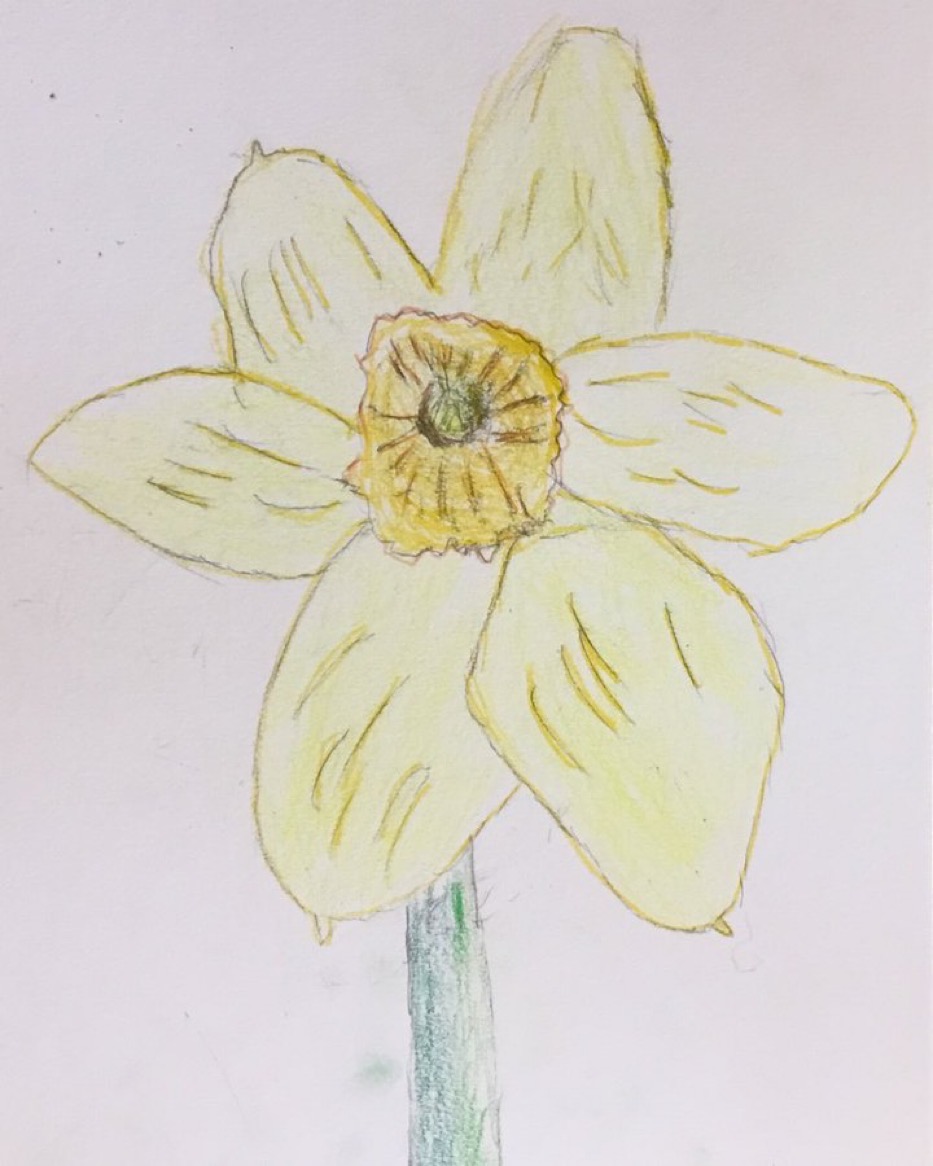The image depicts a colored drawing of a flower, seemingly rendered with colored pencils and outlined in pencil. The flower features a thick, dark green or bluish-green stem with filaments extending from it. It boasts six large yellow petals that extend outward. The center of the flower is detailed with an uneven, bushy yellow bulb containing a smaller dark brown circular shape. Radiating from this dark brown center are long brownish-black lines. A black sprout appears to extend from the green center. The flower is set against a light pink background within a square box, with small black dots visible in the top left corner. The artwork lacks an artist's signature.